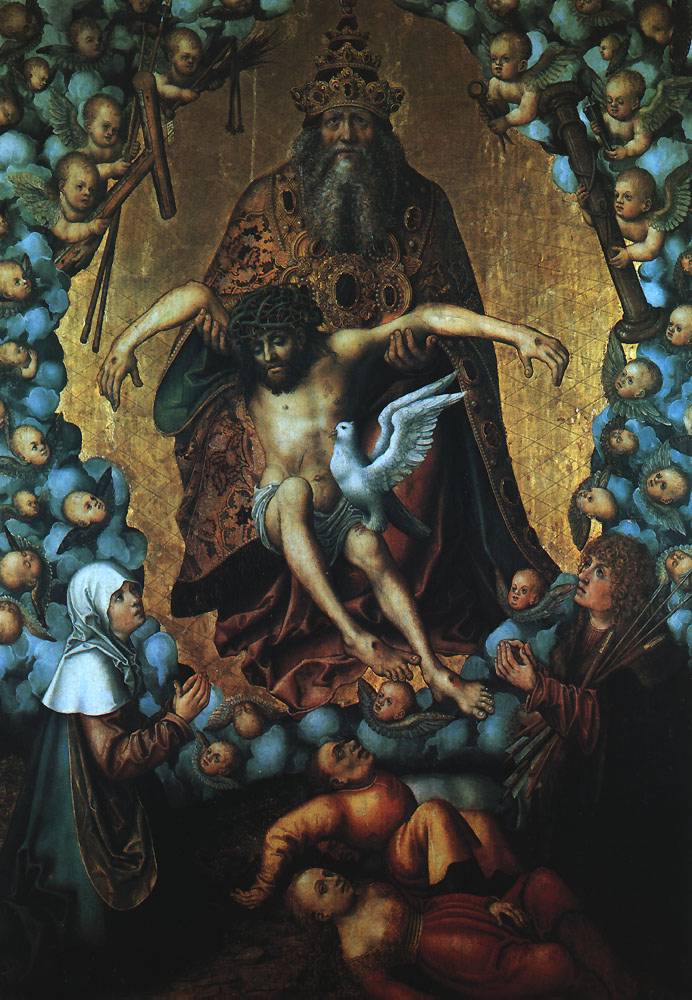This renowned Renaissance oil painting from the 1500s, titled "The Holy Trinity," vividly represents the Christian belief in the Father, Son, and Holy Spirit. At its center, an elderly man adorned in a golden robe and crown, suggestive of divine kingship, cradles a figure commonly identified as Jesus. Jesus is depicted with dark brown hair, a beard, and bearing the stigmata—wounds on his hands and feet and a crown of thorns. A white dove, symbolizing the Holy Spirit, rests on Jesus' knee with its wings outstretched.

Surrounding the central figures, the composition includes numerous cherubs or angelic beings draped in light blue garments, enhancing the celestial ambiance. On the left of the painting, a woman in a white veil and brown robe kneels in prayer, while on the right, a man with brown hair similarly kneels, both gazing upward towards the Holy Trinity. At the feet of Jesus lie two figures, likely representing the slain remnants of evil, dressed in varied clothing with expressions of grimace and pain.

This intricate and detailed portrayal of the Holy Trinity, accompanied by the praying figures and the symbolic representation of good prevailing over evil, underscores the deep religious significance and the exquisite craftsmanship of the Renaissance era.